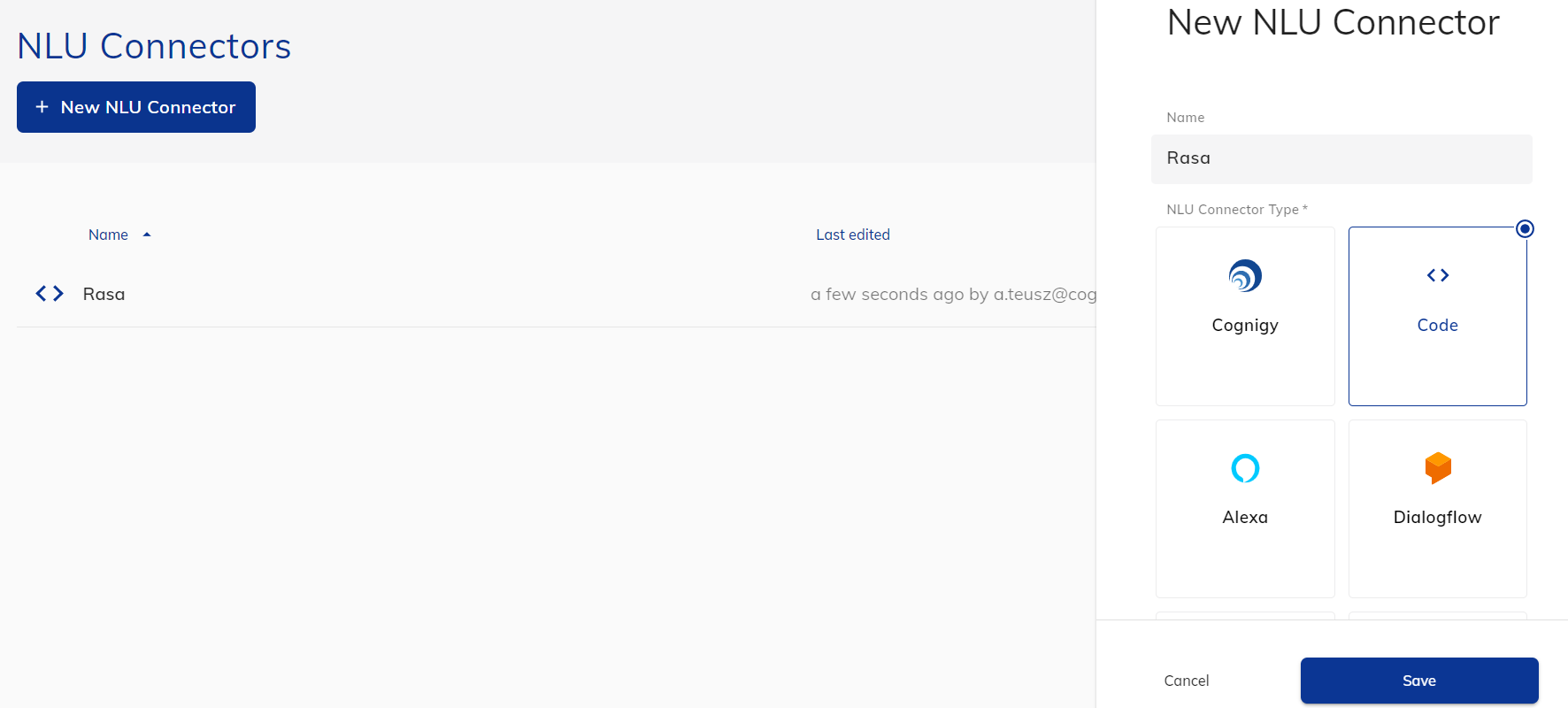The screenshot captures the interface of a device screen showcasing the "NLU Connectors" section. At the top left corner, the screen prominently displays "NLU connectors," followed by a clickable option labeled "+ New NLU Connector." Directly below, there is a sortable column heading named "Name" with an upward arrow indicating sorting criteria. Adjacent to it on the right, there is another column titled "Last Edited."

In the main body of the interface, you can see an entry with "Rasa" (spelled R-A-S-A) listed, accompanied by two arrows—one pointing left and the other right—beside the entry. Further down the same row, it notes "a few seconds ago by A.T-E-U-S-Z," followed by a cutting-off cog icon. This entire section is visually distinguished by a grayish rectangular background.

To the right of this gray rectangle is a white background area where the user is prompted to create a new NLU connector. Here it says "New NLU Connector" at the top. Below, it fields "Name: Rasa (R-A-S-A)" and for the "NLU Connector Type," it notes "Cogna Cognity." Additionally listed are other code options like "Alexa" and "Dialogflow." At the bottom of this section, the interface offers two actionable buttons: "Cancel" and "Save," with the latter being a blue rectangular button.